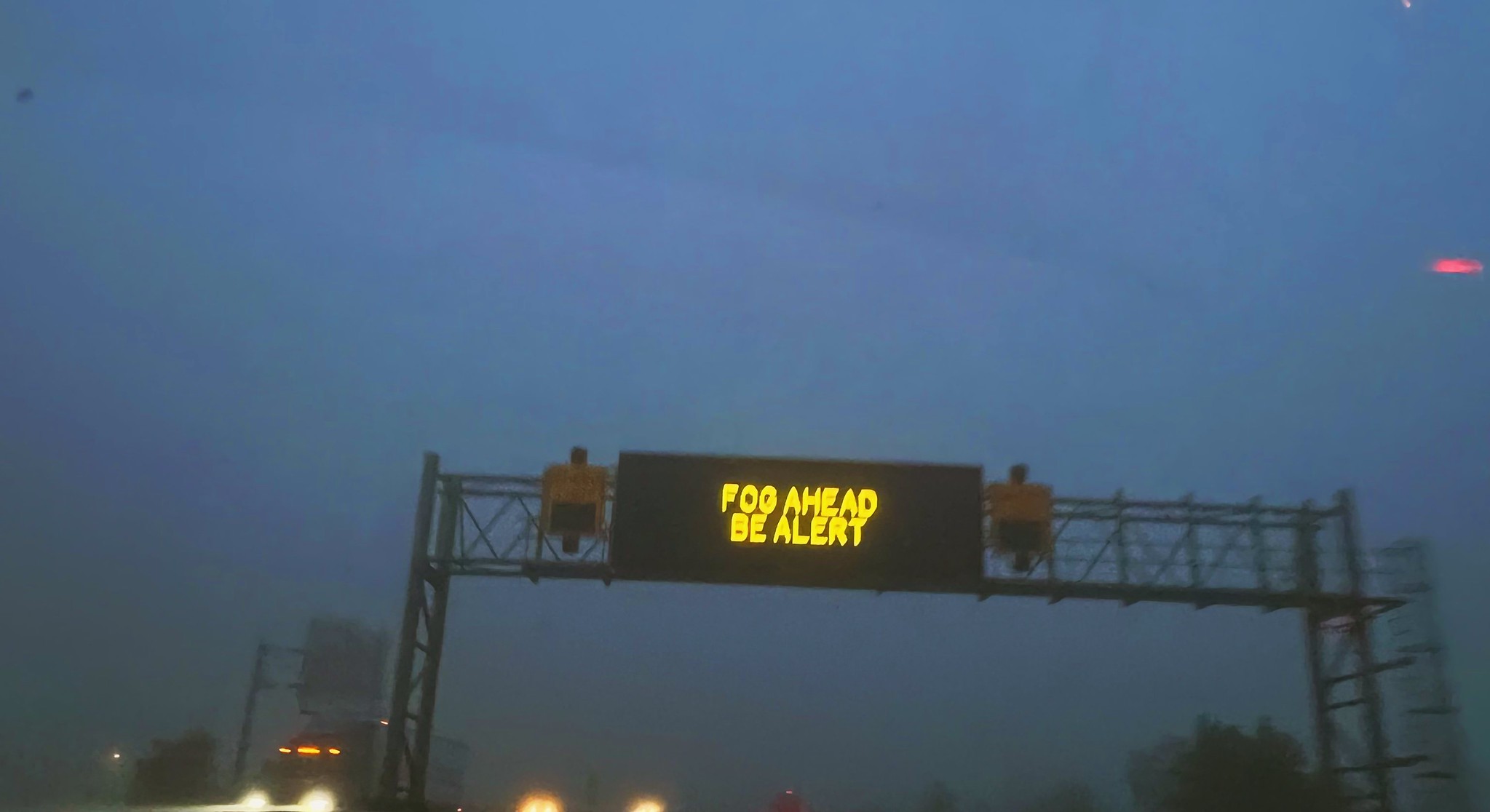This slightly blurry photograph captures a dark, foggy highway scene under a deep blue and purple-tinted sky. Centered in the image is a rectangular digital sign mounted on metal grid work over the roadway, displaying in bold yellow capital letters: "FOG AHEAD" on the top line and "BE ALERT" below it. The sign is easily visible to drivers. Below the sign, the headlights of an oncoming semi truck and some other indistinct vehicle lights are visible, cutting through the murkiness. On each side of the digital sign are two yellow objects, adding to the overall visibility. To the right of the sign, the top of a tree is faintly visible, along with a peculiar pink disc high in the sky. Despite the partial cutoff of the image, the photograph effectively communicates the cautious atmosphere of the foggy road at night.